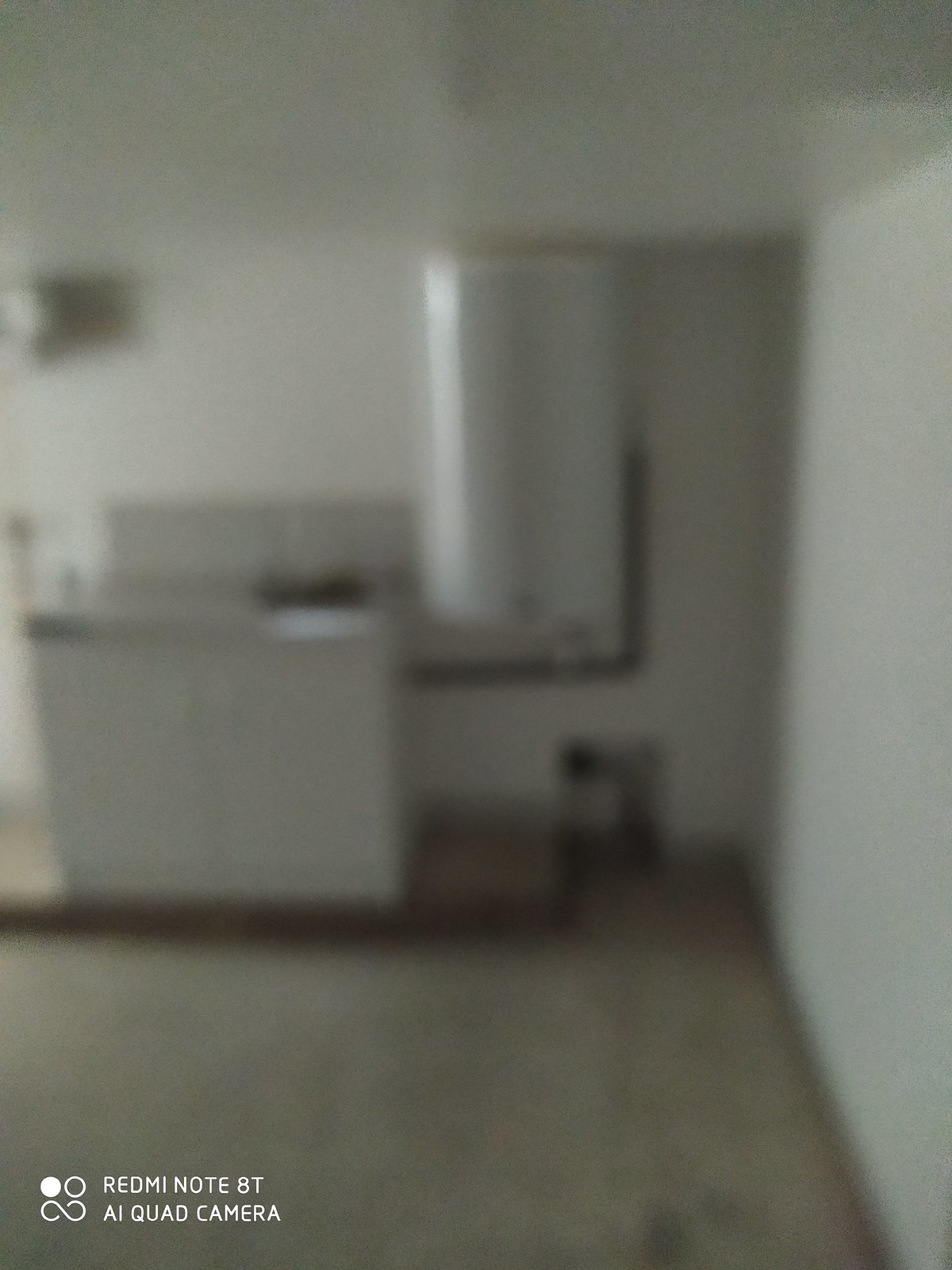The image depicts a sparse room that appears to be a lab or hospital setting. The floor is made of wood or a laminated material resembling wood. The back wall features a countertop with a grey surface, supported by white cabinets below. There's a small backsplash area above the countertop. It is unclear whether a sink is present on the counter. To the right of this setup, a cylindrical object, white in color, is attached to the wall. This cylinder extends from the height of the countertop nearly to the ceiling. Piping or wires emerge from the right side of this cylinder, running down to the floor and then over towards the countertop area. On the floor beneath the cylinder, there is an object resembling a bucket. In the upper left-hand corner of the image, an item protrudes from the wall; it could possibly be a sconce or a light fixture. The overall room is quite minimalistic. In the bottom left-hand corner, there is some kind of symbol next to the text, "README NOT AT AI QUAD CAMERA." The entire background is blurred, adding to the ambiguity of some details.